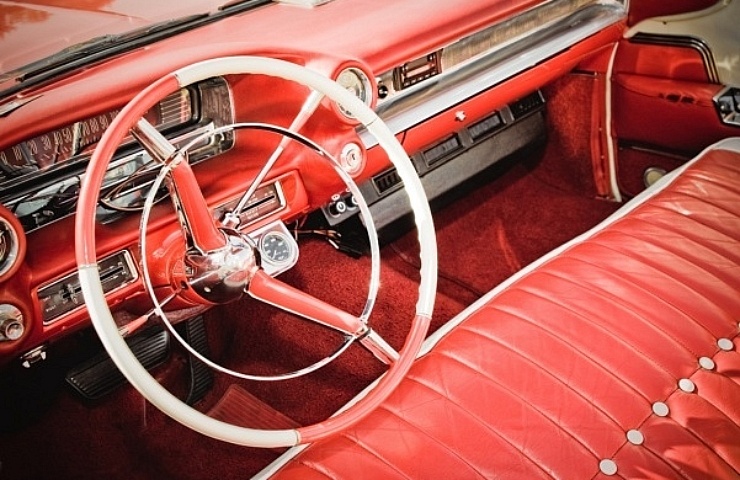This close-up photograph captures the vibrant and meticulously detailed interior of a 1957 Ford Thunderbird convertible with its top down. The focal point is the large, red and white checkered steering wheel with dual red metal bars extending down to the steering column. The dashboard is painted a bold red, adorned with chrome plating around the old-school, retro speedometer and air conditioner vents. On the passenger side, the dashboard features a sleek black radio and a prominently chrome glove compartment. The interior is furnished with a plush red carpet and a matching red leather bench seat, intricately detailed with white buttons running down its center. Visible elements include the black gas and brake pedals, as well as the red passenger side door. The upper left corner of the image even reveals a sliver of the windshield, all contributing to the nostalgic charm and classic elegance of this vintage vehicle's cockpit.